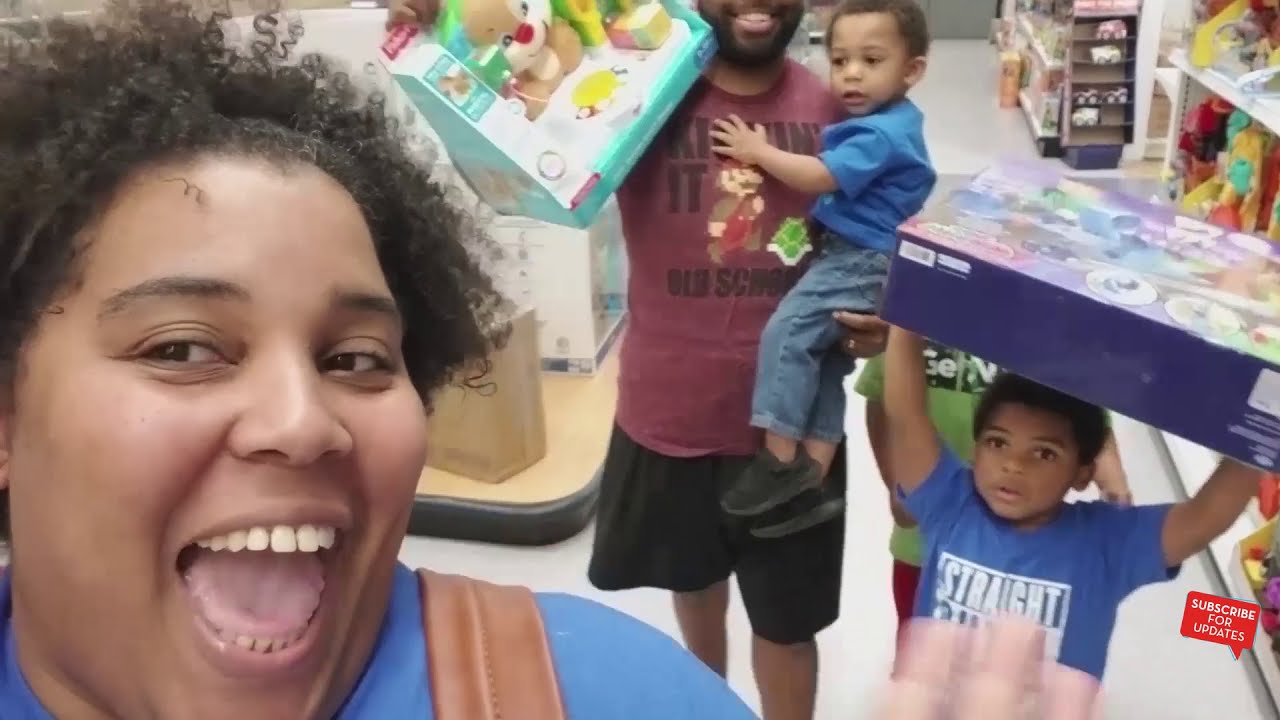In this lively image, an African-American family is captured in the midst of a joyful moment at a toy store, possibly indicating they might be vloggers as suggested by a "subscribe for updates" text on the lower right. At the forefront, the mother is seen with a bright, wide-open smile, almost sticking her tongue out in a playful expression. She’s wearing a blue shirt and possibly a brown bag strap can be seen on her shoulder. Her tight, curly hair is slightly frizzy as she looks at her phone angled towards her, though her gaze is off towards the left instead of the camera lens. Behind her is the father, whose head is partially cut off by the frame. He dons a dark red T-shirt with a pixelated Mario figure and the phrase, "kicking it old-school," along with black shorts. In his left arm, he holds their younger son, a toddler dressed in a blue shirt and jeans, who is gazing to the side with a neutral expression. Meanwhile, their older son, around seven years old, stands nearby holding a large toy box above his head, also outfitted in a blue shirt with white text. The father carries another toy box with a stuffed animal in his free hand, all set within the vibrant aisles of the toy store, adding to the cheerful ambiance of family fun.